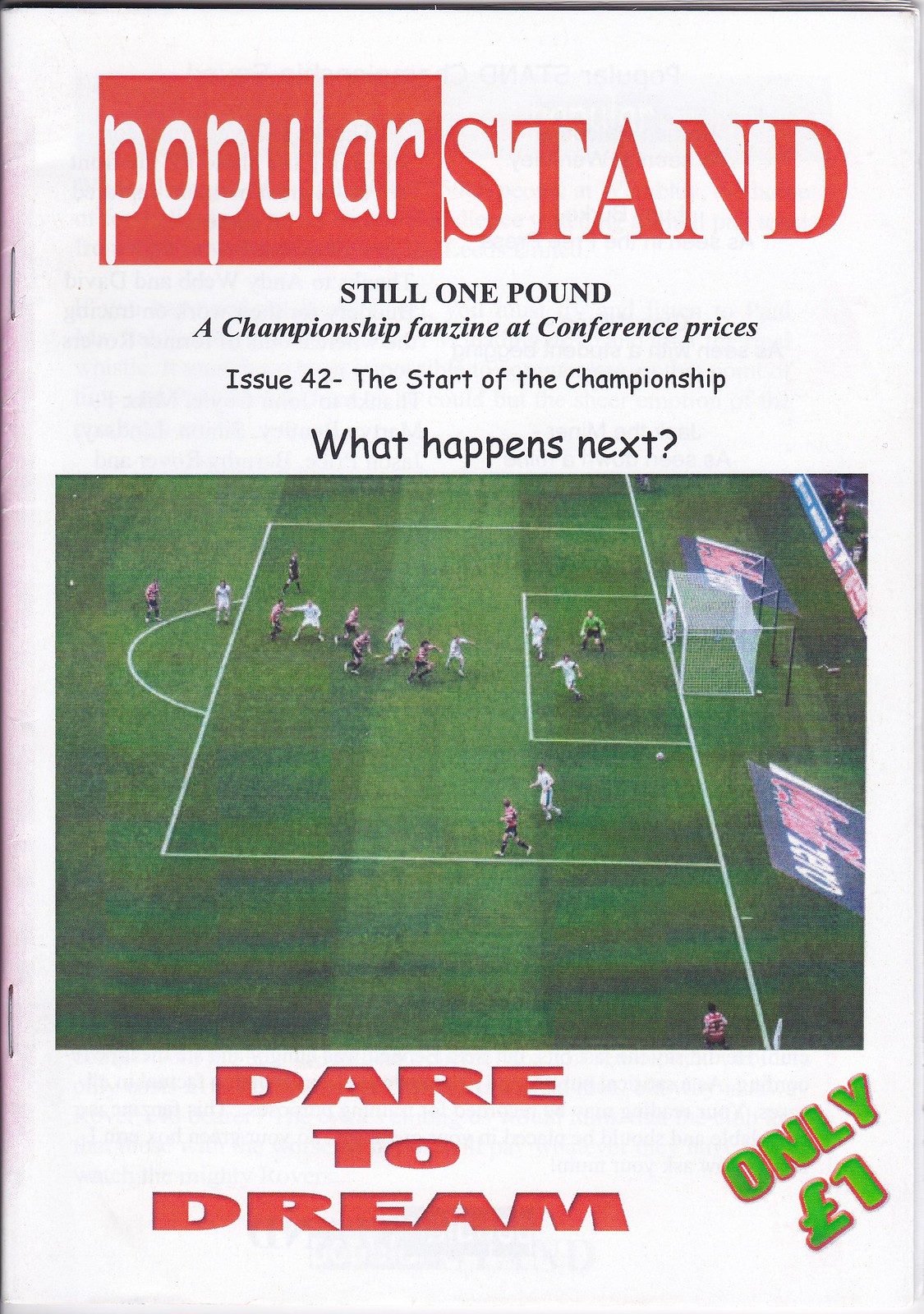The image depicts a magazine cover on a white background. At the top left, there is a prominent red rectangle with "POPULAR" written in white font, followed by "STAND" in bold red capital letters against the white background. Just beneath these, the text "STILL ONE POUND" appears in black font, with the subheading "A championship fanzine at conference prices. Issue 42 - The start of the championship. What happens next?" Below this text, in the center, there's a grainy photograph of a green soccer field taken from above, featuring clustered players near a white soccer net. The bottom section of the image showcases the bold red capitalized phrase "DARE TO DREAM.” Additionally, angled diagonally on the right corner in green font is the text "ONLY ONE POUND." The image effectively combines details about the soccer theme with the magazine's enticing offers and nostalgic touch.